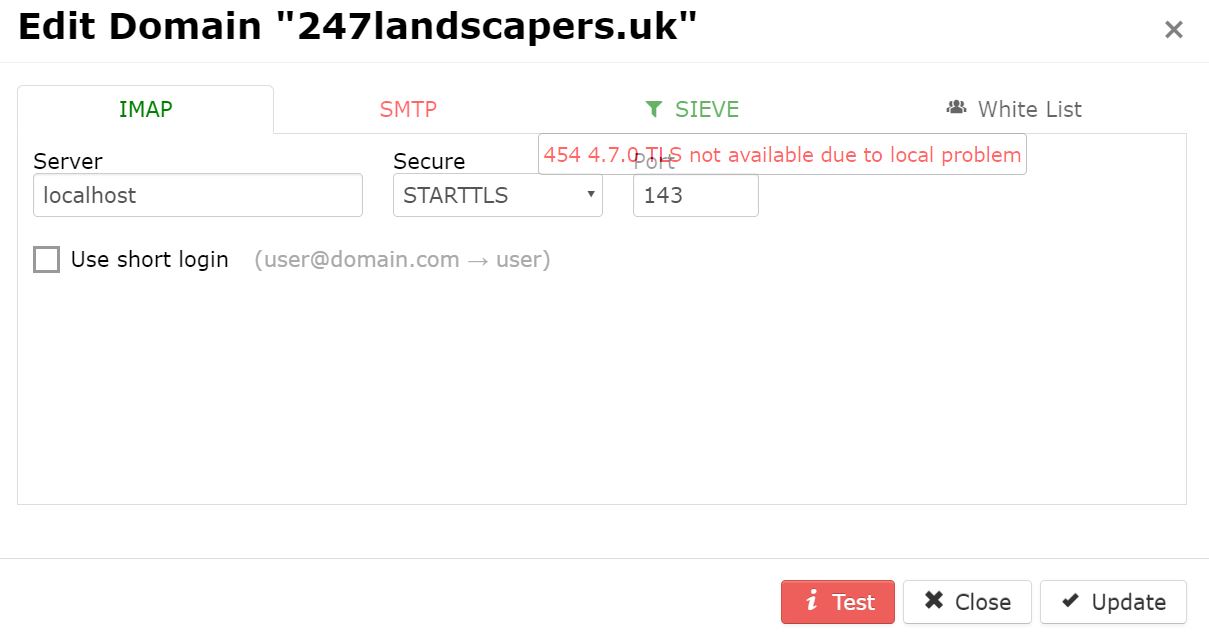The image features a user interface with a white background, prominently displaying "Edit Domain (247landscaper.uk)" in bold black letters at the top left corner. To the top right, there is a gray 'X' icon. Beneath this header is a horizontal light gray line extending from left to right. Below that, the word "IMAP" is highlighted in green letters with a corresponding tab, followed by a section labeled "Server" containing a text box with the placeholder text "localhost." To the right of "Server," there are two labels: "Secure" with a drop-down menu displaying "STARTTLS," and "SMTP" written in red above "Sieve" written in green. Under this section is an error message in red lettering: "454 4.7.0 TLS not available due to local problem." Below this, another text box contains the number "143," and to the right of it is a small label "Whitelist." Additionally, there is an unchecked checkbox labeled "Use short login (user@domain.com)" situated below the "Server" section.